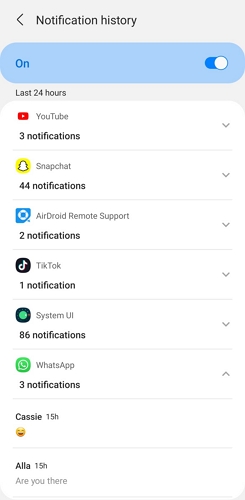The image depicts the notification history screen of a cell phone. At the top of the screen is a gray bar that features a back arrow on the left. Next to the arrow, the text "Notification History" is prominently displayed in black font. Below this header is a toggle switch that is currently in the "on" position, spanning the width of the screen. The phrase "Last 24 hours" appears beneath the toggle.

The main portion of the screen lists notification sources from the last day, divided into eight distinct rows. Each row contains the name of the application along with the number of notifications received:

1. YouTube: 3 notifications
2. Snapchat: 44 notifications
3. Android Remote Support: 2 notifications
4. TikTok: 1 notification
5. System UI: 86 notifications
6. WhatsApp: 3 notifications